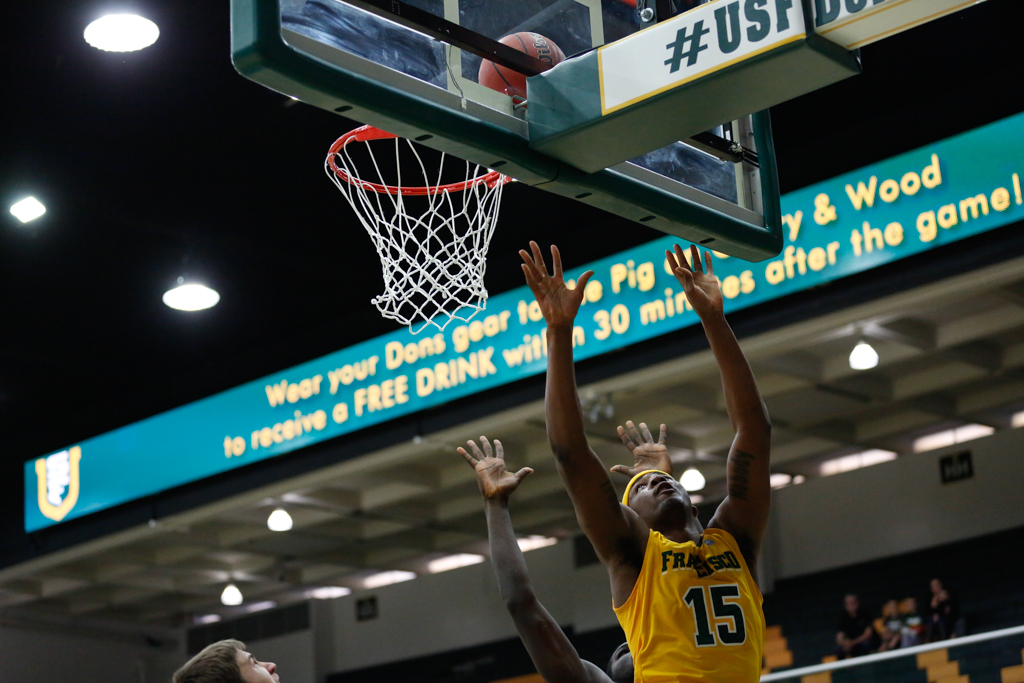The image captures a dynamic moment in a basketball game, focusing on a tall, black player in action. The player, wearing a yellow tank top with the number 15 and a matching yellow headband, is depicted from the waist up with both arms outstretched as he appears to shoot the ball towards the hoop. The basketball is shown just above the rim, indicating either an imminent basket or a rebound attempt. In the background, another player extends his arm, likely trying to block the shot, while a third player’s head is visible, looking up at the ball. The arena's ceiling, with its circular lights, and some electronic signage can be seen, including a blue ad displaying a message about wearing "Don's gear" for a reward at a local eatery. The arena stands are partially visible with a sparse audience, and the overall shot is angled upwards, emphasizing the height and intensity of the action.